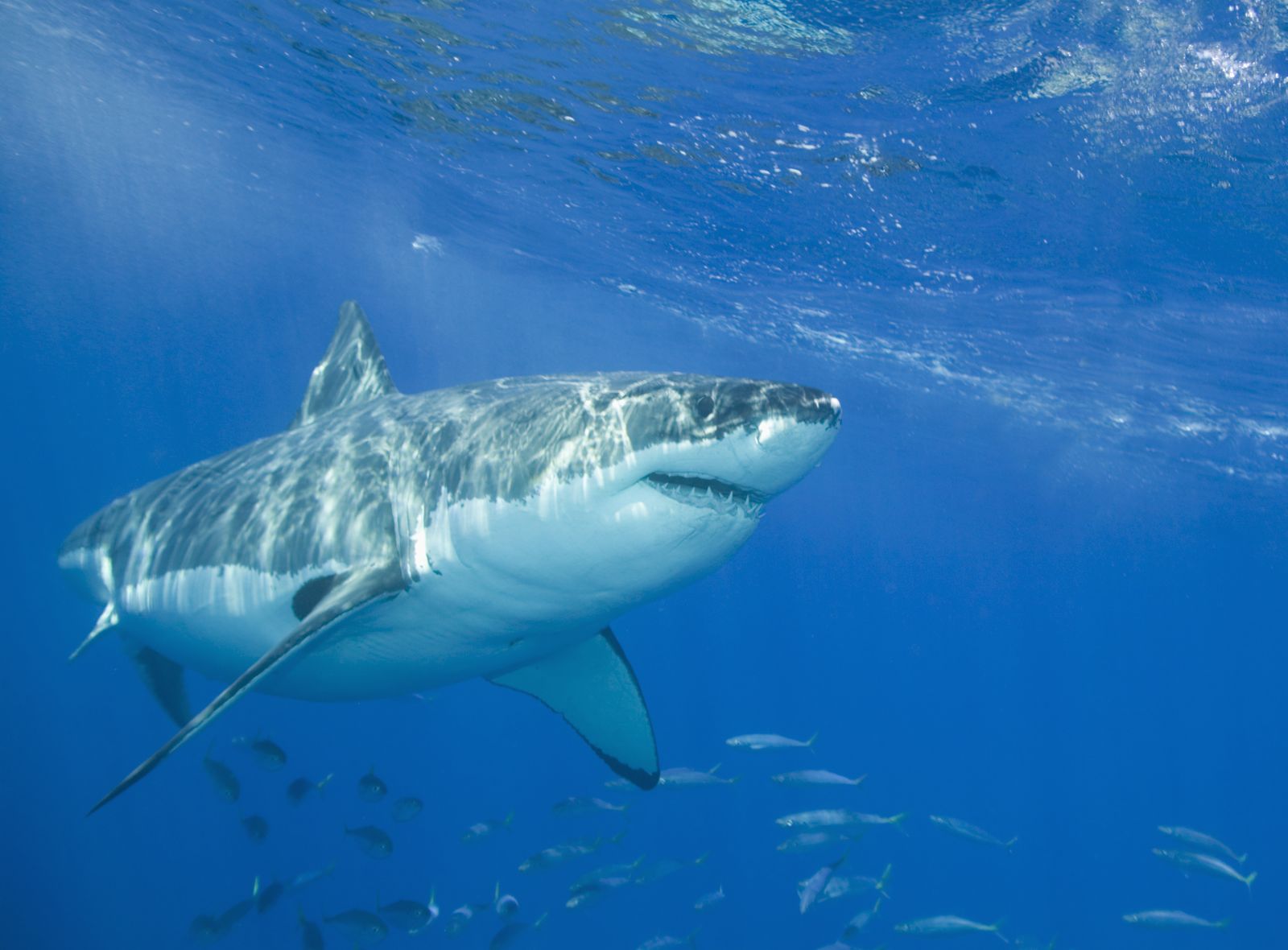This underwater photograph captures a striking scene of a large shark, possibly a great white, swimming close to the surface in beautifully clear, light blue water. The shark is depicted with a white underside and a gray top, with its prominent dorsal fin slicing through the water. Its right eye and sharp teeth are visible, adding to the intimidating presence of this apex predator. The shark is oriented facing the right of the camera, and its tail is swishing to the right as well, reflecting the movement through the water.

Beneath the shark, a school of approximately 20-30 smaller fish is seen, trailing behind as if part of an entourage, likely scavenging for leftover prey debris. The photograph captures fine details such as the surface of the water above, with light reflections and possibly some bubbles, suggesting the shark is not too deep underwater. The colors dominating the image are varying shades of blue, gray, and white, contributing to a serene yet haunting underwater scene devoid of human presence, boats, or text. The overall image conveys both the beauty and the menacing nature of marine life in their natural habitat.